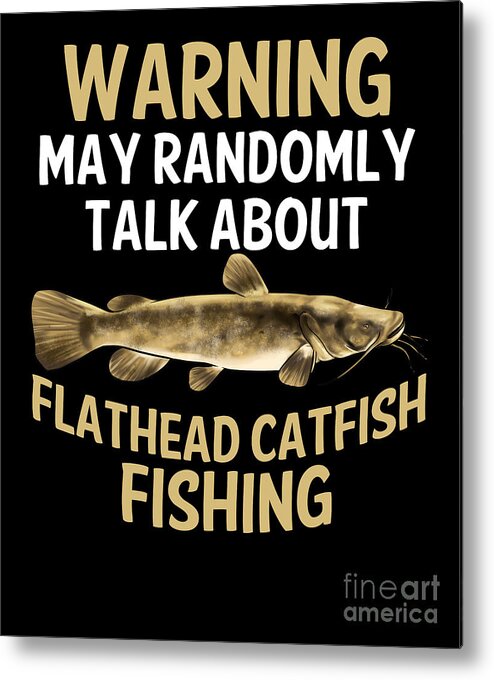The image features a visually striking sign set against a completely black background. At the top, large tan letters in all caps read "WARNING," followed by white all-caps text stating "MAY RANDOMLY" and "TALK ABOUT." Dominating the center is a detailed, brown flathead catfish illustration, complete with distinctive whiskers, a sandy-colored belly, and varying shades of brown and black blotches along its back. The fish's anatomy is precisely depicted, showing the top fin, tail, two side fins, a fin underneath, and a fin near the gills. Below the catfish, more tan, all-caps text reads "FLATHEAD CATFISH FISHING." In the bottom right corner, subtle gray lowercase text says "fine art America." This sign would make an ideal gift for enthusiasts of flathead catfish fishing, perfect for display in a workshop.